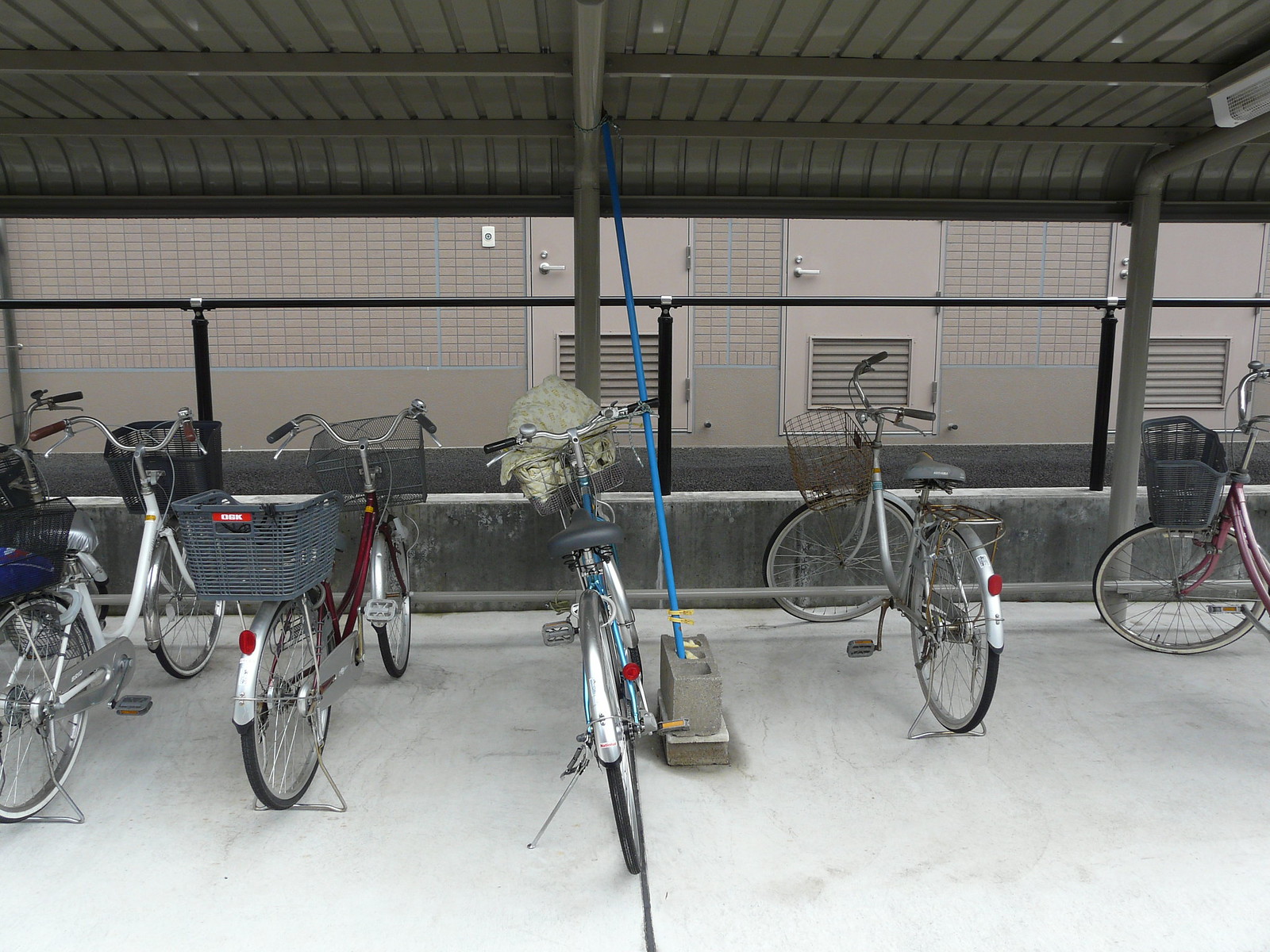This photograph captures a bicycle shed with a corrugated metal roof, viewed from the underside, showcasing its distinct pattern, two sets of support beams, and a gutter. Below, on the concrete base, are five bicycles, with only parts of two additional bicycles visible. These bicycles, ranging from blue, red, white, and pink, are older, commuter-style models, most equipped with baskets either in the front, back, or both. They are neatly spaced apart, each standing on their kickstands. The backdrop features a wall of a building, which includes three metal doors with vents at the bottom, reflecting a dirty grey hue. Surrounding the shed is a mix of metal fencing and a stone retaining wall. There’s also a notable blue pipe inserted into a cinder block. The color scheme of the shelter includes dark green iron steel sheets and support pillars, contrasting with the cream-white brick wall. This visually rich scene potentially depicts a bicycle parking area at a school, station, or office block.